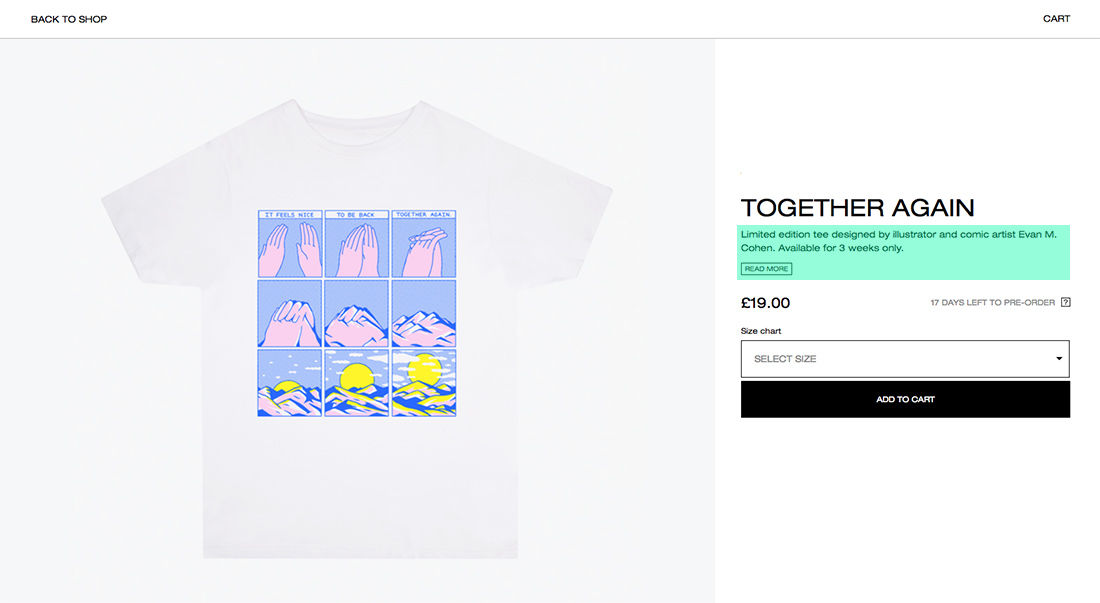This image is a screenshot of an online clothing website that specializes in selling uniquely designed shirts created by various artists. At the top left corner, there is a "Back to shop" button in black text, suggesting that users can navigate back to the main shop page. On the top right corner, the "Cart" icon, also in black text, indicates where users can view the items they have added to their shopping cart. Currently, there doesn't appear to be any items in the cart as no numerical indicator is displayed.

The focal point of the screenshot is a detailed depiction of a white t-shirt located at the bottom left of the screen. This t-shirt features a captivating comic panel design presented in three horizontal rows. The design showcases a transformation theme, starting with a disjointed hand in the top left panel. As the sequence progresses, the hands draw closer together, eventually morphing into a majestic mountain shape. From this mountain, a vibrant sun emerges, creating a visually appealing and cohesive artwork that transitions from seemingly unrelated elements to a unified, stunning image.